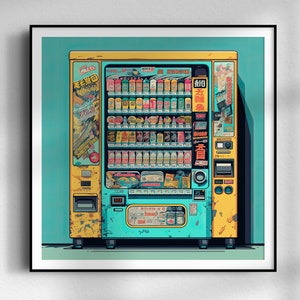The image displays a detailed artwork of a vending machine set against a light blue background, possibly transitioning to teal, with a lighter blue or grayish floor. The artwork is encased within a black square picture frame with a white inner border, all set against a stark white wall. The vending machine itself is visually striking with its metal body, featuring a yellow border on both sides and the top, while the central section is blue or teal in color. It is intricately detailed with several ports, buttons, and display graphics on both the left and right sides, utilizing a palette that includes black, gray, white, red, orange, yellow, and blue. The machine is stocked with six horizontal rows of variously colored products, suggesting high-tech elements reminiscent of advanced vending machines commonly found in parts of Asia, particularly Japan.